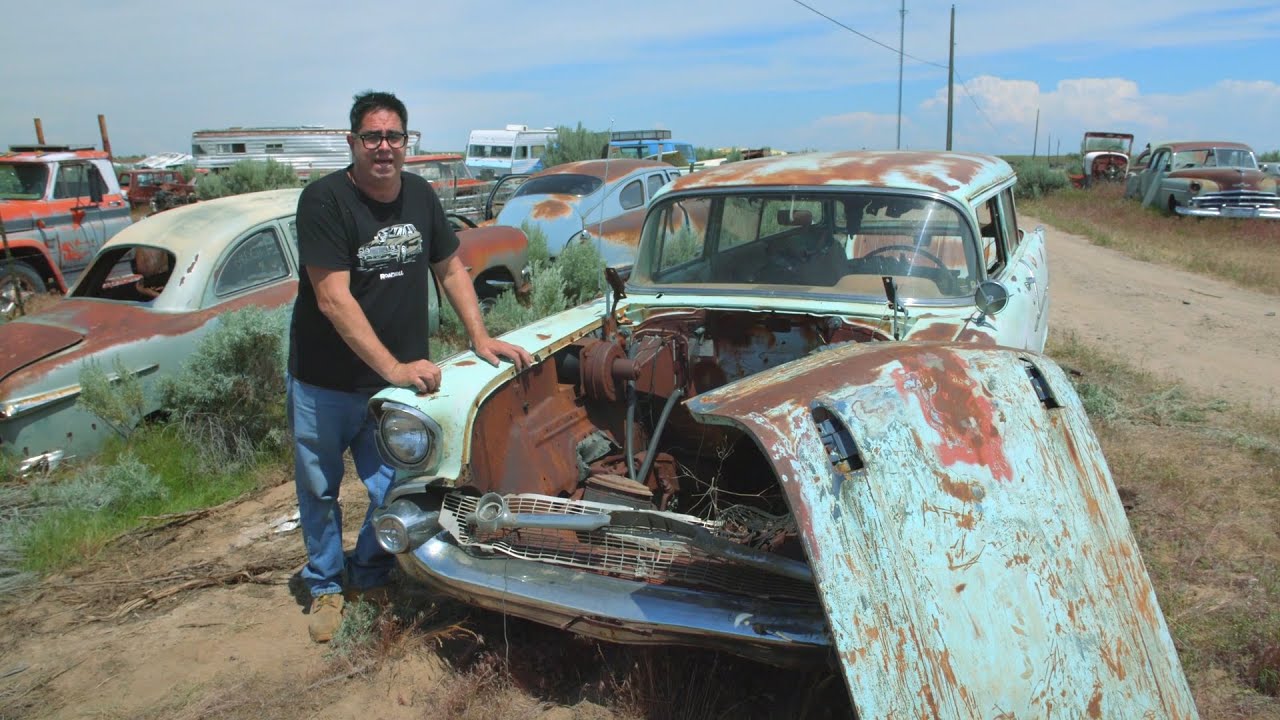In a sprawling junkyard filled with an assortment of rusted and distressed vehicles from decades past, a man stands next to a particularly dilapidated teal car, now mostly a rusty brown hue due to extensive chipping and corrosion. The car, notably missing its hood, exposes an empty engine compartment. Its body showcases thick chrome bumpers and extra-large headlights—design elements that harken back to a bygone era. Peering through the windshield, the car's large steering wheel and hard leather seats are visible, with the driver's side window notably absent. The surrounding area is cluttered with more broken-down cars, a few RVs, and various other vehicles in similar or worse conditions. The man, sporting a black t-shirt with a car graphic, jeans, tan shoes, and glasses, is leaning against the car, looking at the camera without a smile. He stands amidst the relics under a sky dotted with scattered clouds, embodying a poignant scene of automotive history left to rust.